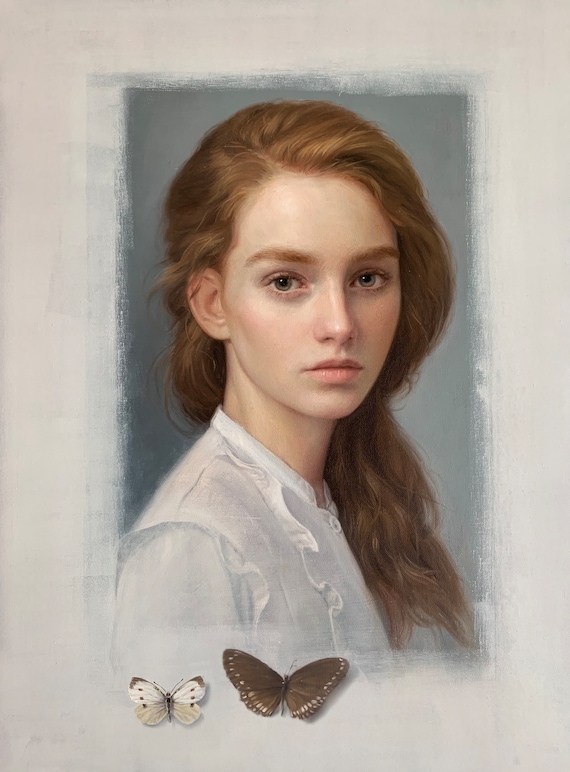This contemporary portrait painting depicts a young Caucasian woman with a red complexion and long, thick red hair cascading behind her head and over her right shoulder. She has striking brown eyes and thick eyebrows, with light pink lips and a faint blush on her cheeks. Her expression is somber and serious. The woman is wearing a white button-down shirt adorned with ruffles on the sleeves and front. The painting showcases a two-tone background: a deep-ish gray rectangular area immediately behind her, framed by a tan outer edge. Below her portrait, two butterflies are depicted—one predominantly white with brown dots on the left, and the other brown with white dots on the right. The entire painting is surrounded by a rough-edged white border, giving it a framed appearance. There are no visible signatures from the artist to identify who created this evocative piece.